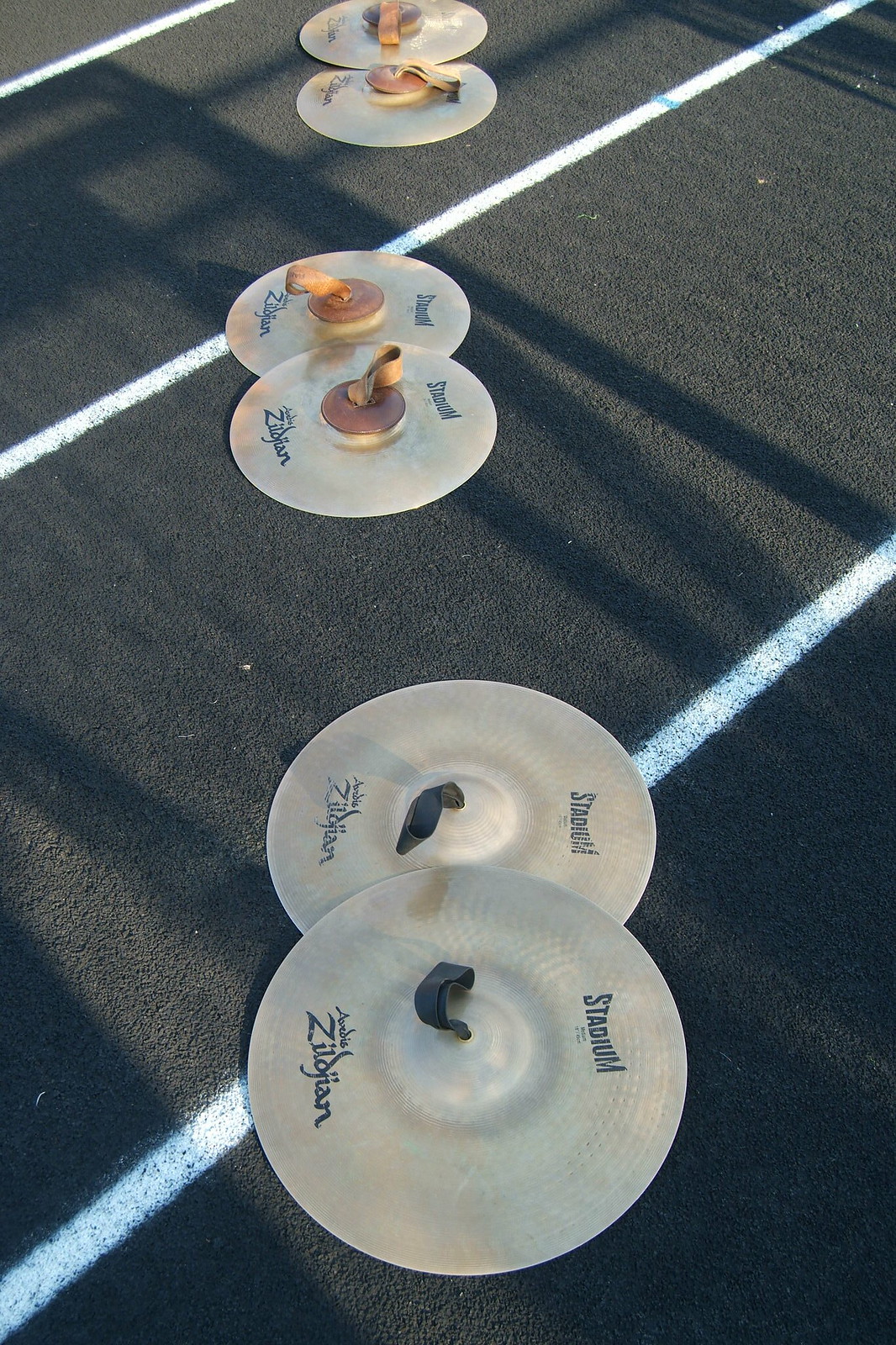This photograph captures three pairs of Zinjian brass cymbals laid flat on a black asphalt parking lot. The parking lot backdrop features white diagonal lines stretching from the top right to the bottom left. The cymbals, resembling round, flat wheels, have smooth, light brown metallic surfaces. Each pair is positioned along a central vertical line from the bottom middle to the top middle of the image. The cymbals, resting at the lower foreground, feature black straps and inscriptions with "stadium" text at the top and "zoo John" at the bottom. Further up, the middle cymbals share a similar design but have brown straps. The topmost cymbals are partially obscured by shadows, making the text less legible. Shadows cast diagonally across the image, hinting at structures like pole silhouettes, add depth to the scene.